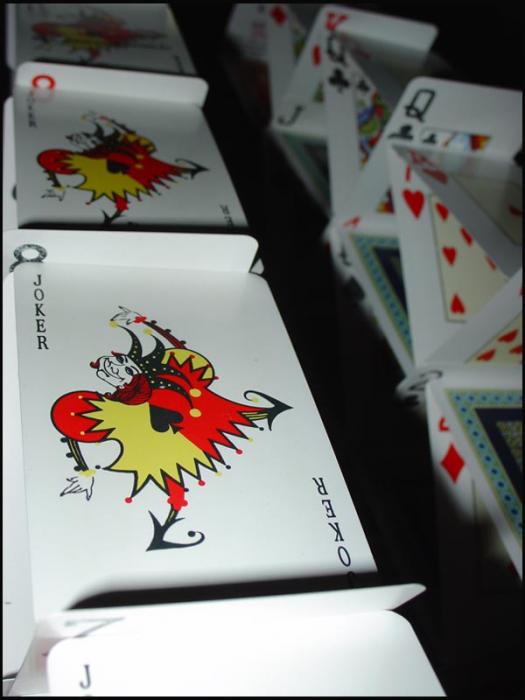The image features a uniquely stacked arrangement of playing cards. On the left side of the image, there is a series of Joker cards prominently displayed. Each Joker card is predominantly white with black print that spells out "JOKER" in the upper left corner and identically upside down in the bottom right corner. The central illustration on the Joker card depicts a court jester dressed in a vibrant red and white outfit. The jester has their right arm raised, left arm positioned behind their body, right leg lowered, and left leg raised. Their attire has alternating colors for the shoulders and shirt halves: one shoulder is red and the other yellow, and vice versa for the shirt. A spade symbol adorns the middle of the jester's shirt, and they are shod in black shoes with curly, pointed tips.

This front Joker card dominates the left side, with the numbers 7, 8, and 9 subtly peeking out between the cards in the center top left portion of the image. On the right side, more playing cards are meticulously stacked, creating an intriguing pattern. The arrangement consists of a mix of flat cards, some positioned at a diagonal angle, with others interspersed and standing upright at the ends.